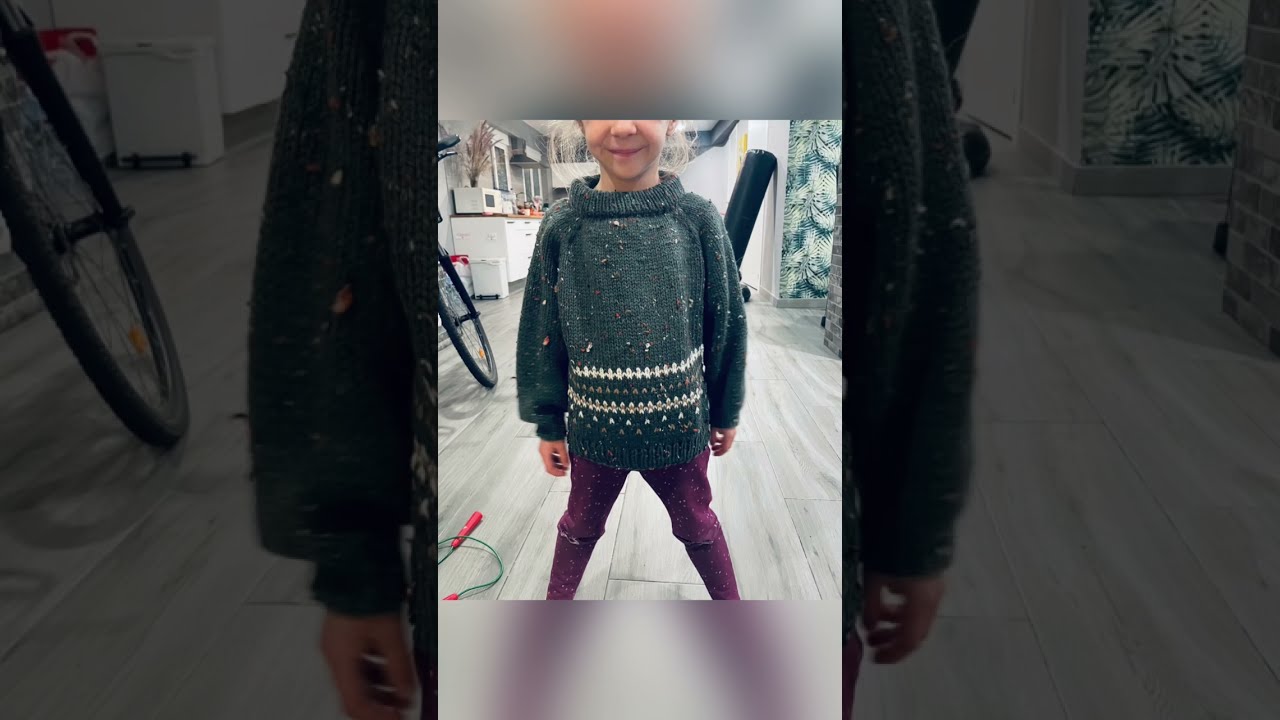In this composite image, a small Caucasian girl stands in a kitchen, her portrait prominently displayed in the center against a blurred, gray, and transposed background featuring an extended landscape view of the same scene. The image is cropped just below her nose and above her ankles, making her smile partially visible. She wears a fuzzy green turtleneck sweater adorned with white stripes and diamond patterns around her waist and long sleeves, paired with crinkly purple pants that may have tears near the knees. The kitchen setting is detailed with a white counter holding a microwave, surrounded by white cabinets and a silver vent hood. To her left is the front tire of a bicycle, and a jump rope lies curled on the wood-patterned floor. The overall scene presents a cozy domestic environment, capturing a moment of playful innocence.